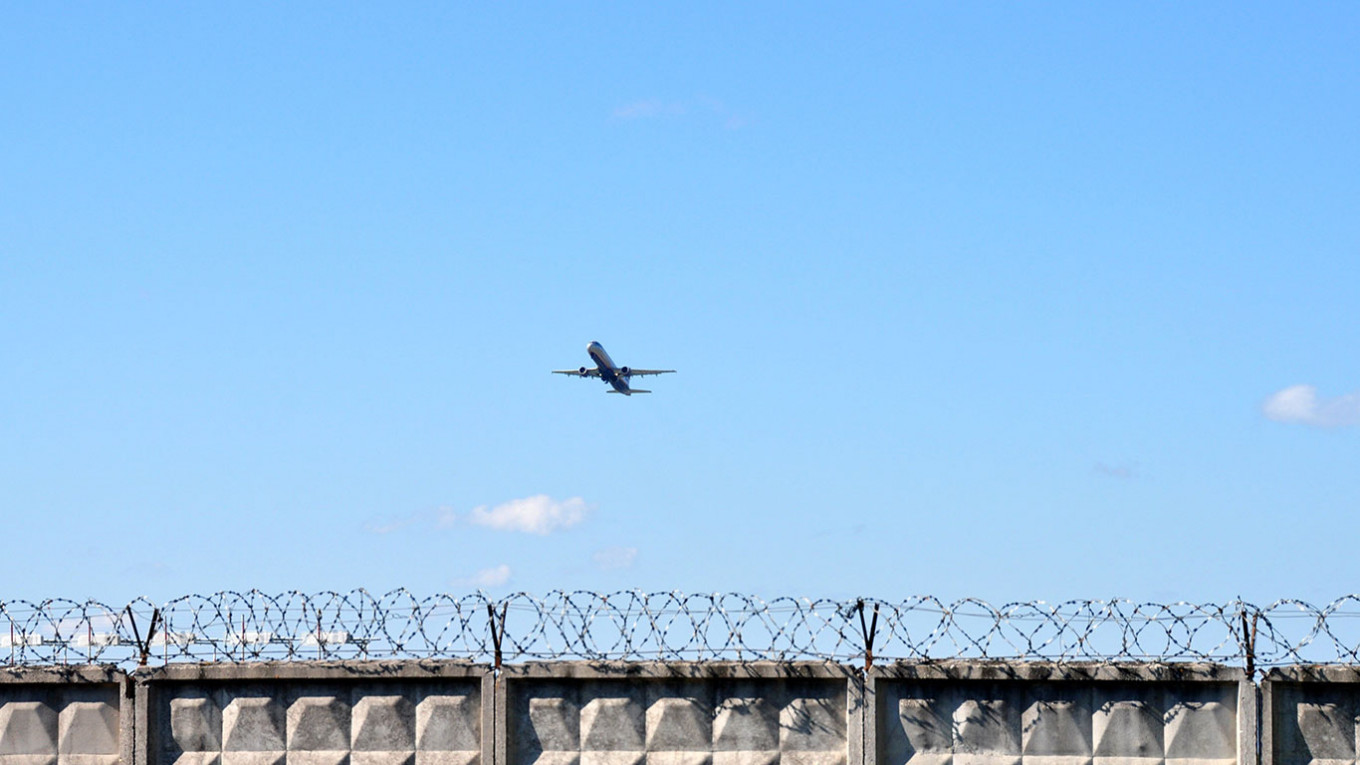The image is a rectangular landscape photograph, wider than it is tall, depicting a vivid scene. The photograph captures a small airplane in mid-flight, positioned centrally and facing diagonally toward the top left, suggesting forward movement. The sky is a brilliant clear blue with a gradient that transitions from a deep blue at the top to a lighter hue at the bottom, punctuated by a few tiny clouds, with one notably to the airplane's bottom left.

Dominating the bottom part of the image is a formidable fence, constructed of gray stone slabs and topped with menacing, circular barbed wire rings, evoking the impression of a high-security area such as a prison. The barbed wire extends across the entire width of the photo, reinforcing the sense of confinement below the open expanse of sky and the aircraft above. The stark contrast between the boundless sky and the restrictive fence highlights the tension within the scene.